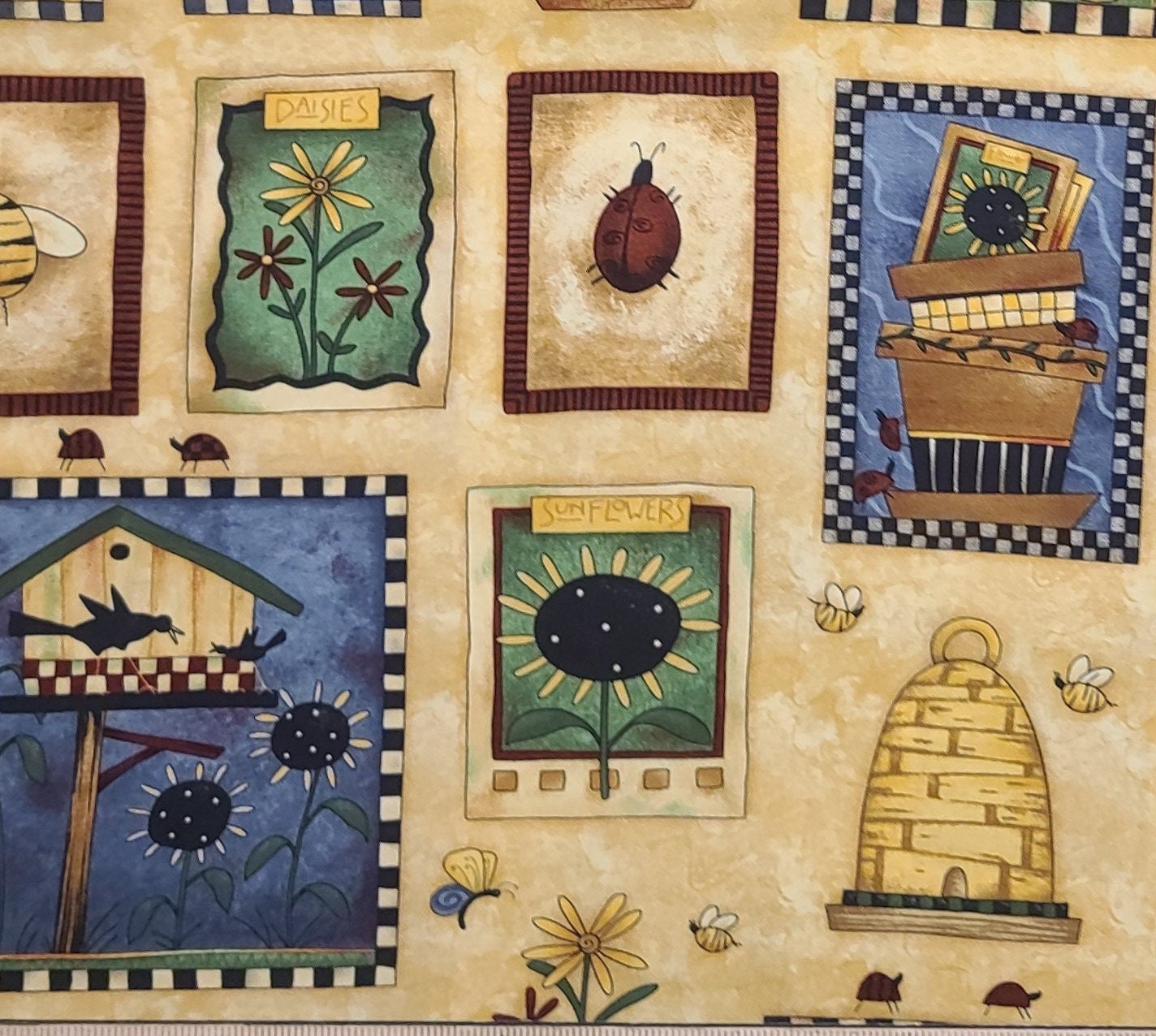The image features a hand-drawn tapestry with a golden brown, parchment-style background with white marbling. Scattered across this backdrop are framed cartoon-style illustrations of various nature scenes, each "photo frame" integrated into the fabric like snapshots of outdoor life. The scene in the bottom right showcases a floating beehive surrounded by playful bees, and nearby, two ladybugs rest on the ground. A sunflower with a butterfly flitting about appears to the left. Above this, there's a collection of other nature-themed illustrations: a bee, a trio of red and yellow daisies in a green frame labeled "daisies," and a ladybug framed in brown. Among these drawings is a distinctive black and white checkerboard frame with a planter displaying another framed picture. A birdhouse on a stick, surrounded by two spiky flowers of varying heights, is also depicted in a blue checkerboard frame. Notably, an image of a vibrant yellow sunflower with a black and white center, set against a green background with a white frame, sits in the top left corner.Adjacent to this, a larger, striped photo frame houses a photo of the night sky with sunflowers and crows. This detailed tapestry, though a bit blurry, represents a charming collection of nature-themed cartoons and frames, giving the feel of a whimsical, hand-drawn gallery woven into fabric.